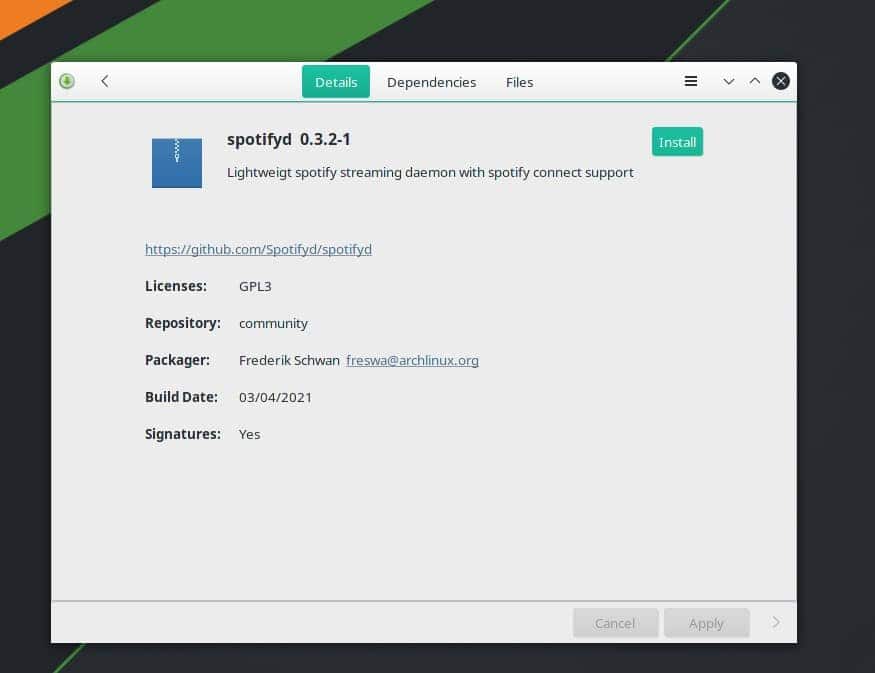This screenshot showcases a pop-up text box with a very light gray background. The backdrop of the image is an abstract design featuring black, green, and orange hues. At the top of the text box is a banner with a green "Details" button, alongside small black text that reads "Dependencies and Files". There are icons situated in the top left and right corners. Below the banner runs a very thin, light green line.

At the center is an icon depicting a blue square with a zipper down the middle, representing a compressed file. Below this icon, the text reads "SpotifyD 0.3.2-1". Accompanying this is a description: "Lightweight Spotify Streaming DAEMON with Spotify Connect support."

Further below, a green "Install" button is positioned above a support link. The link, underlined, directs to "https://github.com/".

The bottom section of the text box presents detailed information in bold black text. The fields listed are:

- Licenses: GPL-3
- Repository: Community
- Packager: Frederick Schwan (with an email link)
- Build Date: 03-04-2021
- Signatures: Yes

In the lower right corner of the text box, there are "Cancel" and "Apply" buttons with a gray background.